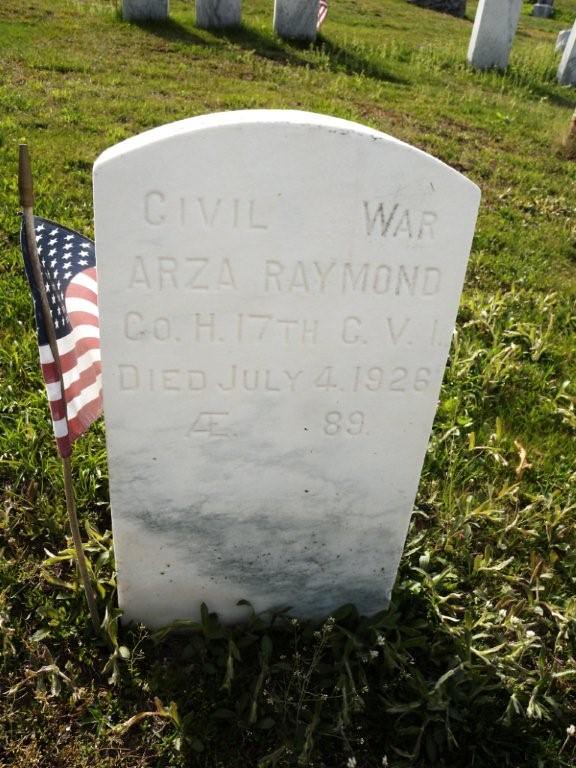This photo features a white marble Civil War gravestone amidst an overgrown cemetery. The gravestone, inscribed with "Arza Raymond, Co. H, 17th, C.V.I., died July 4th, 1926, A.E. 89," stands prominently in the foreground, slightly stained with black smudges at the bottom. An American flag on a small pole is positioned to the left of the gravestone, indicating recent recognition despite the unkempt surroundings of weeds and grass. The cemetery is dotted with several other similar white gravestones, many facing away with unreadable inscriptions, one of which also features an American flag. The scene suggests a resting place primarily for military personnel, marked by simple, uniform headstones amidst a backdrop of green grass and small white flowers. The overall atmosphere conveys a sense of historical reverence albeit with a hint of neglect, as indicated by the unmowed grass and lack of recent maintenance.